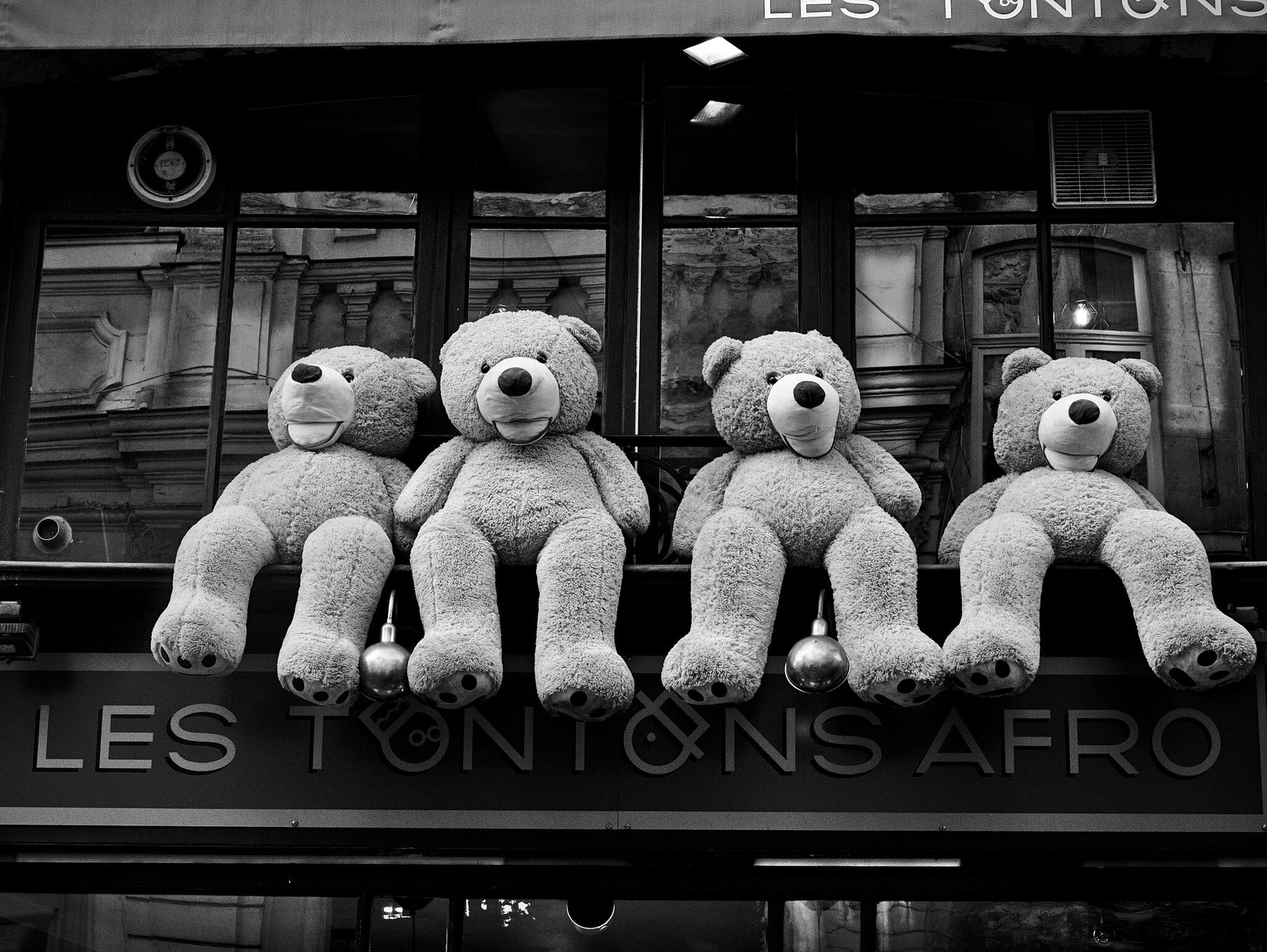In this detailed black-and-white photograph, four large identical teddy bears are prominently perched atop the black overhang of a storefront, legs dangling over the edge. The bears, which are likely a light color such as brown in real life, have noticeable dark noses and eyes, with three distinct round dots on the bottoms of their feet resembling toes. The storefront below their feet features the name "Les Tantons Afro" in French, displayed in silver text on a black background. The overhang also has a light gray strip with cutout white text, partially visible at the top of the image. Behind the bears, several windows reflect a stone building from across the street, adding depth to the photograph. A small Christmas tree bulb is hanging from one of the teddy bears, introducing a whimsical touch to the scene. The entire setup suggests an older, charmingly structured building, with the teddy bears serving as an inviting and playful attraction.